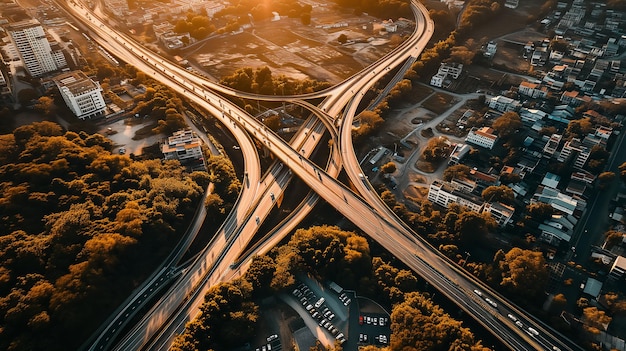This detailed aerial photograph captures an expansive freeway interchange, possibly in the L.A. area, where multiple highways intersect and crisscross in a complex network of roads. The most prominent highways run diagonally from the top right to the bottom left and from the bottom left to the top right, intersecting in the middle. Additional on-ramps and off-ramps spiral around this central intersection, creating a web of connectivity. 

The sun bathes the entire scene in a warm, yellow-orange hue, casting a glow over various features. To the far left, a dense cluster of yellow and green-hued trees creates a natural contrast to the urban environment. The bottom middle of the image showcases a parking lot filled with numerous cars. 

On the far right, a bustling area of a town or city is visible, dotted with houses, buildings, and likely commercial structures such as business buildings or hotels. The upper left corner reveals an apartment complex along with additional buildings and roads, some multi-story and varied in color from white to gray. The photograph provides a detailed and dynamic view of a vibrant mixed-use area, blending residential neighborhoods with commercial zones and significant infrastructure.